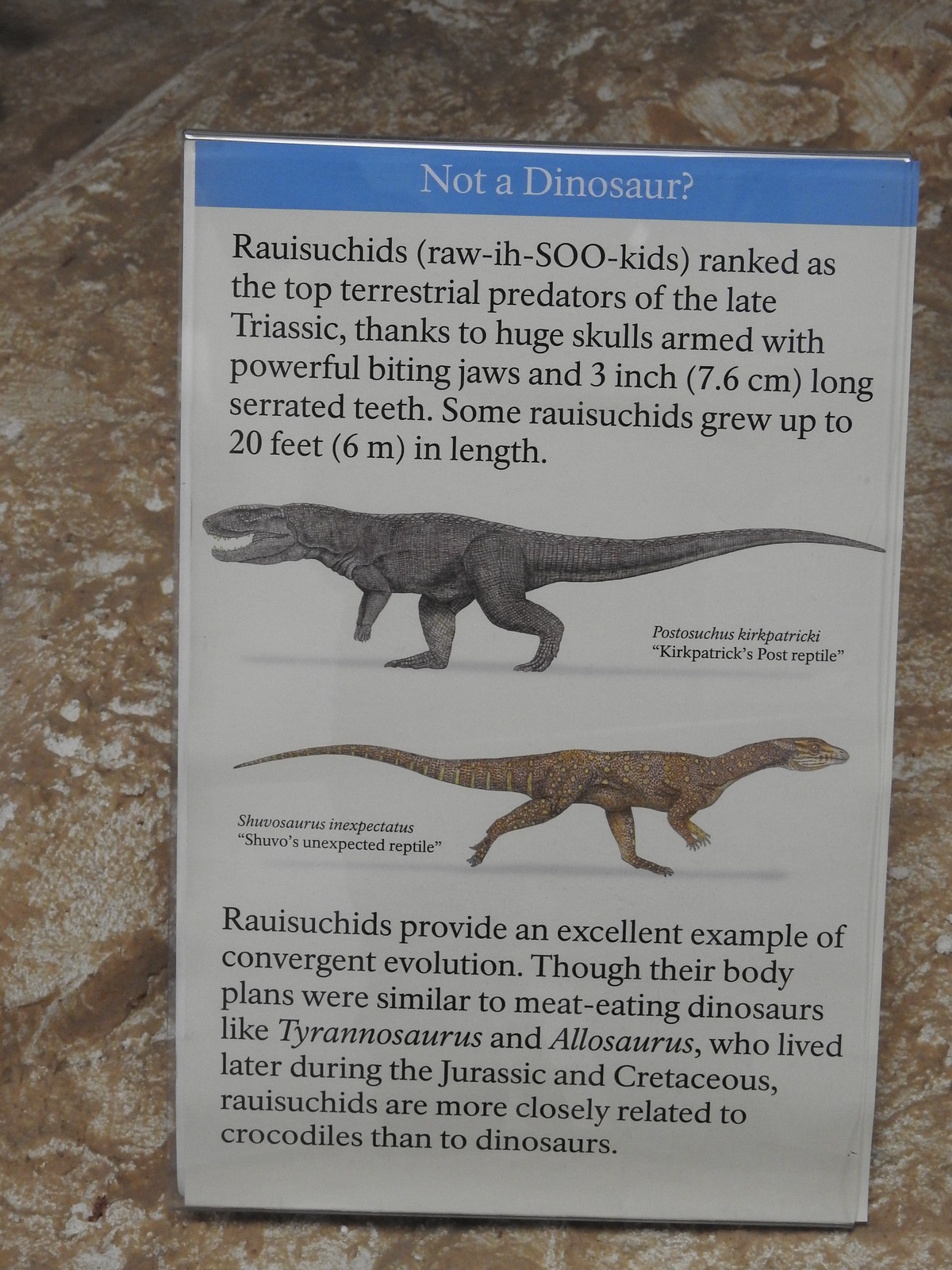This image captures a detailed informational plaque that appears to be either in a museum or placed outdoors, leaning against a beige, white-speckled rock. The rectangular sign with a white background is taller than it is wide, and features a bold blue header at the top, which reads "Not a Dinosaur?" in white text. 

Below the header, the plaque provides an in-depth description of "Rauisuchids" with pronunciation guidance: R-A-W-dash-I-H-dash-capital-S-capital-O-O dash-K-I-D-S. These creatures were the top terrestrial predators of the late Triassic era, thanks to their enormous skulls, powerful jaws, and three-inch (7.6 cm) long serrated teeth. Some Rauisuchids grew up to 20 feet (6 meters) in length.

The plaque includes illustrated images of two Rauisuchid species: a gray-colored Postosuchus kirkpatricki, moving left to right, identified in the lower right-hand corner, and a brown-colored Shuvosaurus inexpectatus, moving from right to left, noted in the lower left-hand corner. Both images highlight their lizard-like appearance.

At the bottom of the sign, additional text explains that Rauisuchids are an excellent example of convergent evolution. Despite their similar body plans to later meat-eating dinosaurs like Tyrannosaurus and Allosaurus from the Jurassic and Cretaceous periods, Rauisuchids are actually more closely related to crocodiles than to dinosaurs.